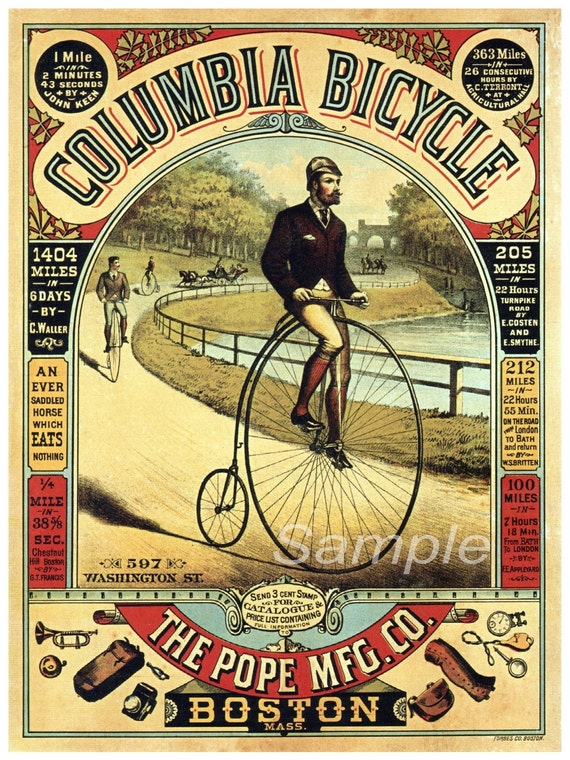This vibrant, vintage advertisement for Columbia Bicycle is designed as a square poster and features a prominent illustration set against a beige background. The banner at the top arches with the bold text "Columbia Bicycle." The scene depicts a man from the 1800s riding a distinctive penny-farthing bike with an oversized front wheel and a tiny rear wheel. He wears a brown hat, a black or brown tuxedo with a black tie, a white undershirt, a white handkerchief in his pocket, beige leggings, and high knee red socks. His distinguished curled mustache and beard complete his look. Behind him, a few other individuals can be seen: two on similar bicycles and one in a chariot drawn by horses, with additional horses and arches visible in the background, along a tree-lined road that leads past a cyan-colored pond.

The advertisement is rich with text and detailed statistics on the bike's performance. Key figures include: "1 mile in 2 minutes and 43 seconds by John Kelm," "363 miles in 26 consecutive hours by C. Trent," "1,404 miles in 6 days," "205 miles in 22 hours," and "100 miles in 7 hours and 18 minutes.” The advertisement also highlights an exceptional claim: "An ever-saddled horse which eats nothing."

In the lower section of the advertisement, there is a black text box with yellow lettering that states, "Boston Mass." Nearby imagery includes a trumpet, a stopwatch, a backpack, a camera, a satchel, and other objects, adding to the period ambiance and appeal of the ad.